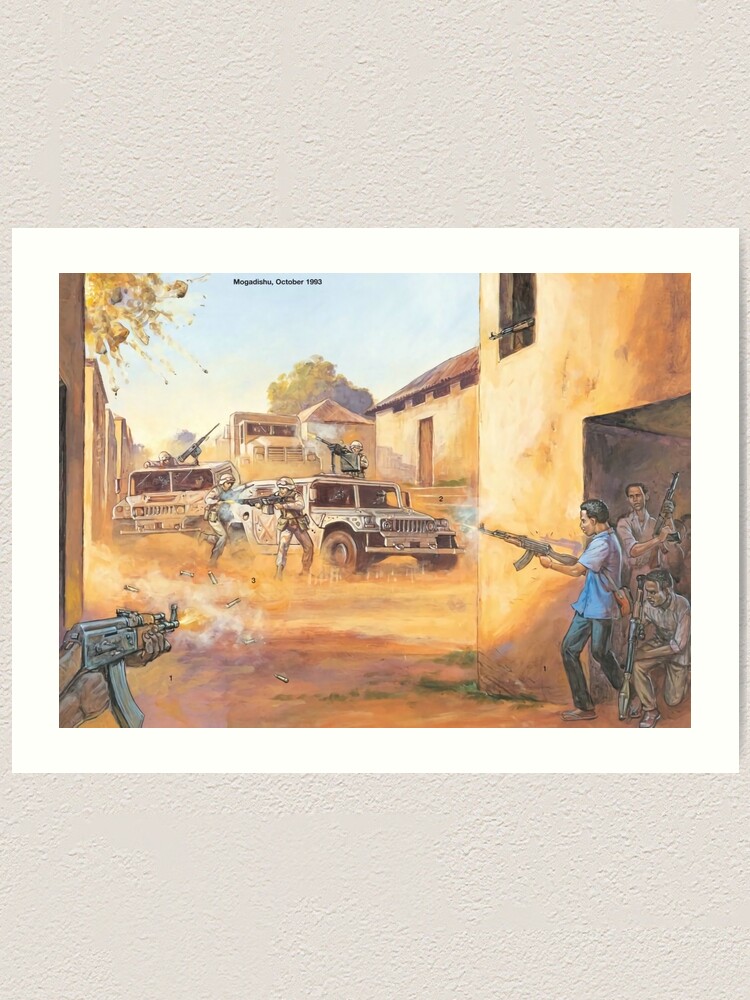The image depicts a war scene set against a white background, presenting a detailed, painted portrayal of the Battle of Mogadishu in October 1993. The setting is a desert-like environment with sandy yellows and tans dominating the landscape. At the top of the painting, the text "Mogadishu, October 1993" is prominently displayed.

In the center of the image, two beige Humvee vehicles are positioned, one bearing a soldier operating a turret gun. Military personnel are scattered around the vehicles, engaging in combat. To the left, a green tree and an explosion can be seen in the background. On the ground, several armed figures—some with AK-47 rifles and one with a bazooka—are positioned in various poses indicative of an ongoing battle.

The foreground reveals more intense fighting: US Marines in the background are firing at hostile forces in the foreground. A concrete or stone building stands prominently with a visible porch and door, flanked by an alley running between two large structures. Men hiding in the doorway are armed, one of whom is firing from an AK-47 rifle towards the military personnel. The vivid storytelling of the painting is supplemented by a blue sky overhead, contrasting the chaotic scene below.